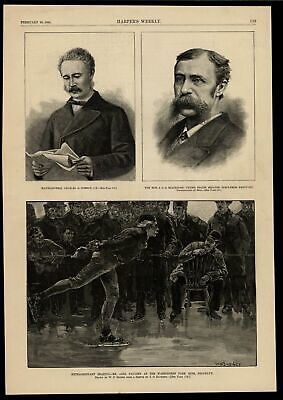The image features a framed, aged newspaper page with a manila, slightly brown color, enclosed in a black border. At the top of the page, there are two illustrated portraits: the left portrait shows a man with a coat, bow tie, and mustache, reading a newspaper, while the right portrait displays another man with thick, bushy mustache, brown hair, and attire consisting of a jacket, tie, and collared shirt. Below these portraits, a large black and white photograph captures a moment of ice skating, where a person glides on the ice with one leg extended behind and arms resting on the small of their back. In the background, a crowd of spectators, many of them wearing hats indicative of an earlier era, watch the skater. The newspaper bears some black text and captions for all the images, although the text is difficult to discern due to its small size and slightly blurred focus. The top portion of the newspaper includes some partially legible words, possibly a title or name, which appear to be "Harfield something."